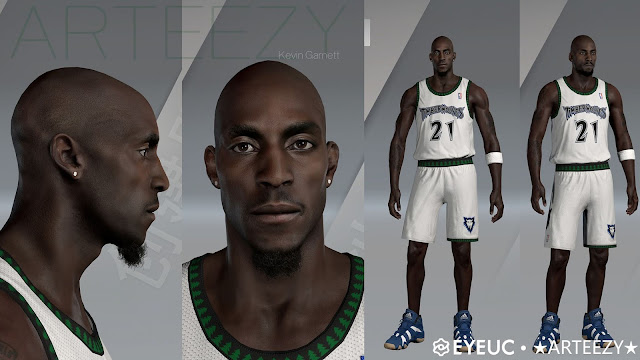This image appears to be sourced from a website and features a collage of four vertical images arranged in a rectangular frame. Each image focuses on a man, likely professional basketball player Kevin Garnett, wearing a distinctive white jersey with green and black accents. 

In the second image, which captures immediate attention, Garnett's dark brown eyes stare directly at the camera. He has a bald head and adorns his ears with diamond stud earrings. A neatly trimmed beard frames his profile. This close-up shot shows him from the chest up, revealing the detailed texture of his jersey and subtly visible green text in the background that reads "Art Easy." Below this text, in bold white letters, is his name: Kevin Garnett.

The first image in the set presents Garnett’s profile, showcasing the same meticulous details of his face and upper torso as the close-up image. 

The third and fourth images shift perspective to a full-body view, where Garnett stands confidently in his complete uniform. The jersey, identifiable by the number 21 in black, pairs with matching white shorts accented with green edges. A logo resembling a wolf, indicative of his team—possibly the Timberwolves—adorns his shorts. He sports blue, white, and cream-colored athletic shoes, and wears a white armband on his left arm. In one of these snapshots, Garnett faces forward, making direct eye contact with the camera, while in the adjacent image, he turns his gaze to the right, adding a dynamic visual shift to the collage.